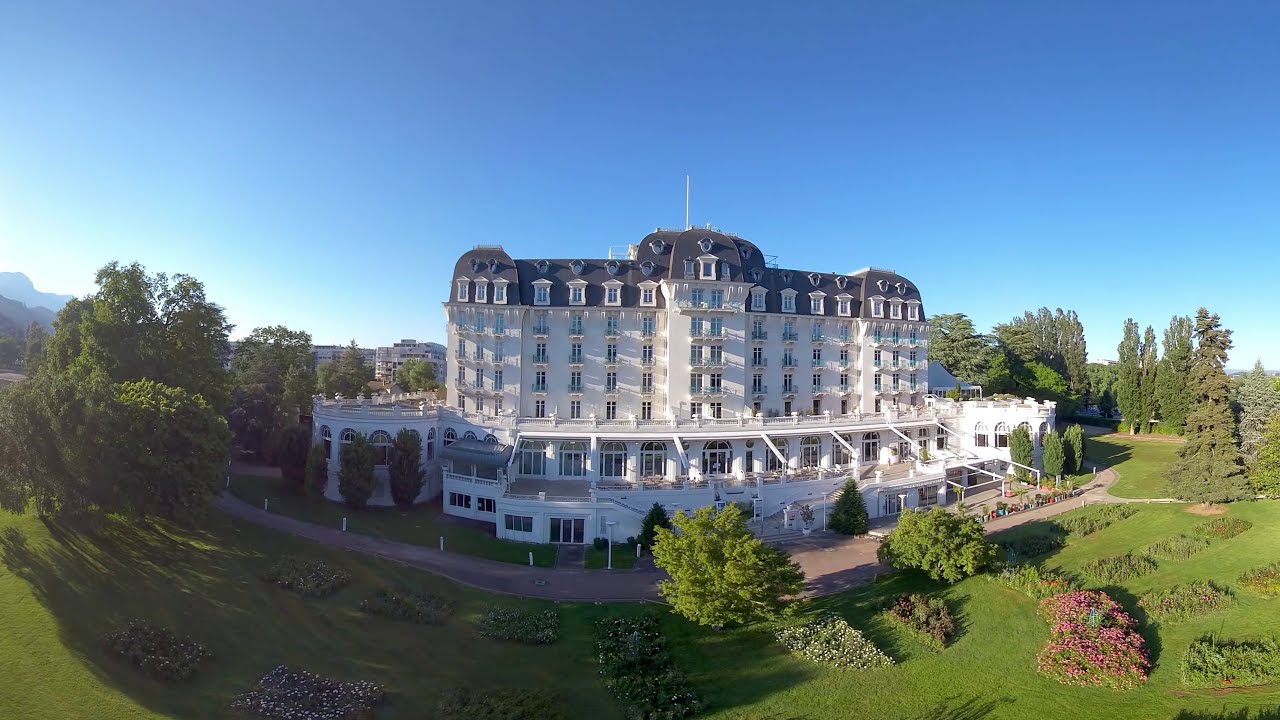This is an aerial, high-quality, 360-degree panorama view of a large, luxurious, white, multi-story building, possibly a hotel, mansion, or castle, with a black or dark gray roof. The building features Neo-Romanesque windows and dormer windows on the top floors, with distinct projecting edges, towers at the corners, and larger bottom floors that jut out from the upper stories. Surrounding the building is a meticulously maintained landscape, including a broad concrete walkway lined with gardens and beds, leading to a sprawling ornamental garden filled with bright green grass, low-lying flowers, well-trimmed shrubs, and vibrant vegetation. The scene is bright and clear, captured during a sunny day with a vivid blue, cloudless sky. The building sits in a secluded area bordered by tall trees, with rolling hills and a hazy horizon visible in the background, adding to the scenic and tranquil atmosphere.